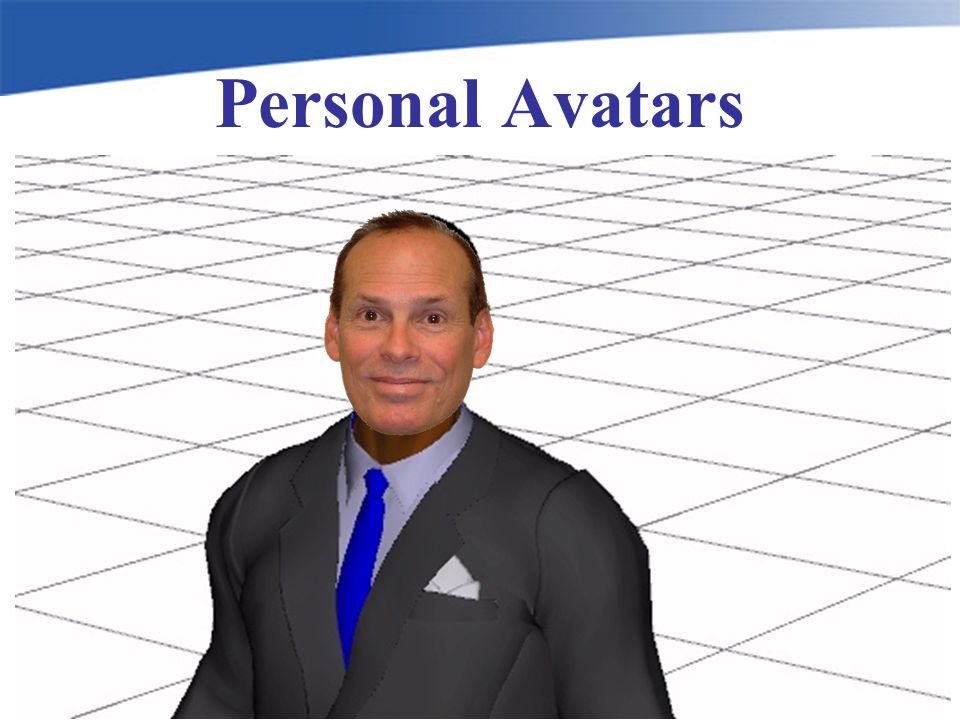The image appears to be a screen grab or PowerPoint slide with a white background overlayed by a black checkerboard pattern. At the top, there is a small blue arc that sweeps from the upper left-hand corner and fades to the right. Below this arc, the phrase "Personal Avatars" is prominently displayed in large blue font, with each word capitalized. Centered in the middle of the image is a computer-generated picture of a man. He is depicted wearing a gray suit, complete with a white handkerchief in his left breast pocket, a light gray button-up shirt, and a dark blue tie. The man's face appears to be an actual photograph superimposed onto the computer-rendered body. He has short dark hair with a receding hairline, brown eyes, a large jaw, and big oval ears. His skin tone is Caucasian or very light brown, and he is smiling with his mouth closed. This detailed and layered composition almost makes it appear as if the photograph was placed over the background.